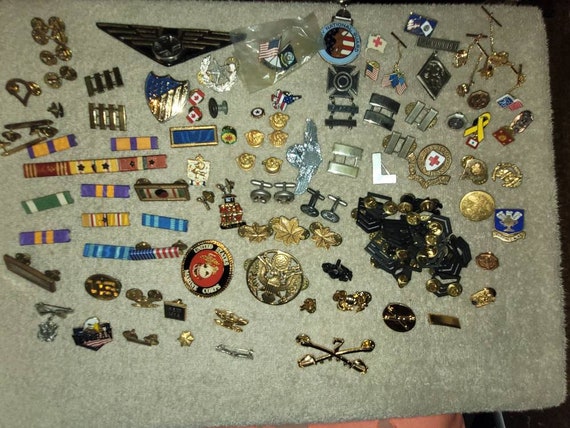This photograph showcases an extensive and meticulously arranged collection of military ribbons, medals, pins, and cufflinks displayed on a gray carpet background. The arrangement features over four dozen individual pieces, with an array of colorful ribbons—yellow, blue, green, white, red, black—which signify various awards and honors. Key items include: several silver and gold pins, some resembling tracks, others in the shape of wings, and a prominent gold ring with a red cross superimposed on a white shield. Notable among the medals is one with two crossed swords and the number seven above it. The collection also contains numerous American flag pins and gold and silver buttons, some emblazoned with an eagle. On the right side of the display, a white "L" stands out, along with a medical symbol featuring a red cross on a white and gold shield. Various other intricate emblems, such as stars, flowers, and additional shields, enrich the assortment, highlighting the diverse and significant accomplishments of the collector.